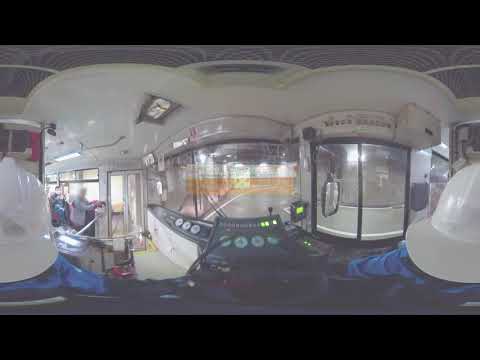The image captures a panoramic view inside what appears to be a high-tech bus or control center. The bus driver, positioned centrally, is dressed in a long-sleeved blue jacket and a distinctive white helmet with a large rimmed back, resembling a fireman's helmet. They have both black-gloved hands on a black steering wheel. The control panel in front of the driver is detailed with various green LED lights, radio monitors, numerous gauges, and levers. 

The bus's interior is predominantly white, featuring a white roof and flooring. On the left side, there are white folding doors with glass panes. Through the large front windscreen, the setting appears to be indoors, as an indoor building is visible outside, suggesting the bus is inside a larger facility.

To the right of the driver, a small pull-open window set in a black frame adds another detail to the control area. The image conveys a futuristic and industrial feel, with the possibility that the bus might act as a control center within a manufacturing or production facility. The panoramic aspect of the image causes some warping, adding to the complexity of identifying precise function but enhancing the detailed portrayal of the high-tech and controlled environment.